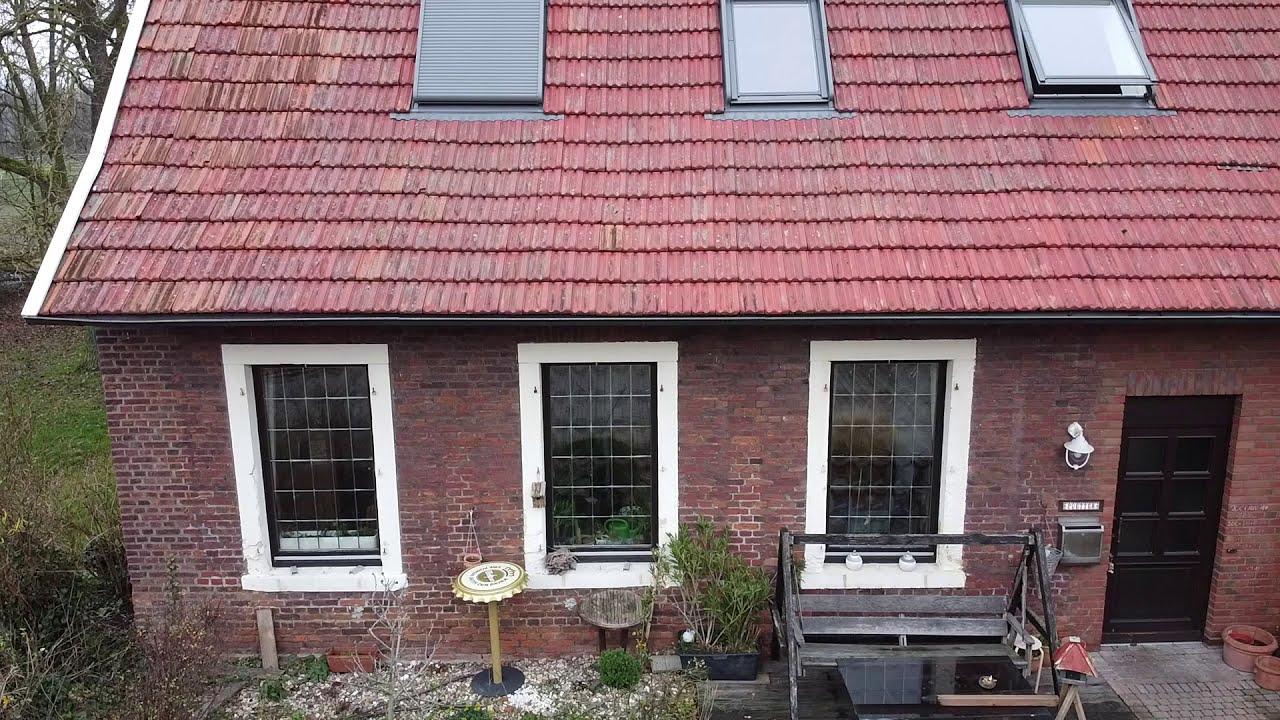The image depicts a quaint red brick cottage, seemingly styled with elements hinting at it being outside of America due to its architectural features. The home has a charming red terracotta tile roof adorned with three large skylights. Three substantial windows, framed intricately in white and divided into about 20 small panes each, are prominently featured at the back of the house. To the right side, there's a door with potted plants beside it on a cement walkway, though the pots appear empty. Adjacent to the door, a mailbox and a light fixture are mounted on the wall. The yard showcases a mix of elements, including remnants of white rock flower beds, suggesting they were once vibrant but now fallow. Of notable interest is a bench swing situated near the first window, and another item resembling a bench swing or possibly a barbecue without cushions. The setting is cluttered with various plants and objects, alluding to an unkempt garden. The left edge of the image reveals a grassy patch with some trees in the background, enhancing the home's secluded and serene ambiance.